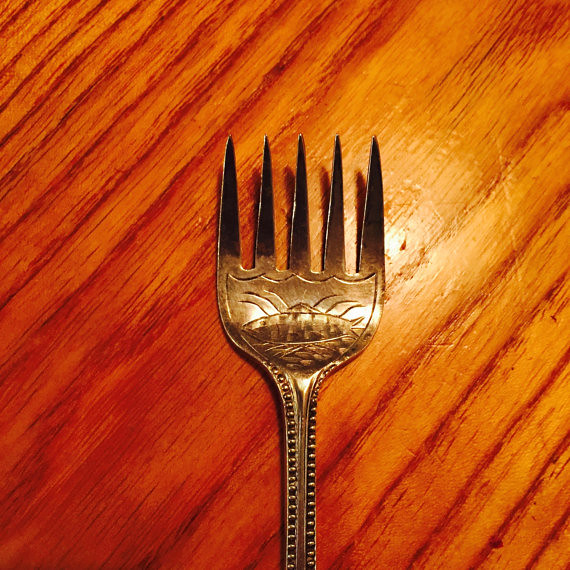This detailed photograph showcases an ornate, antique stainless steel fork with an unusual five-pronged design, lying flat on a light brown wooden surface with visible wood grain. The tines of the fork are notably short and sharp. Below the prongs, the scoop part of the fork features an intricate etched design depicting a fish, accompanied by curved marks above and scales or water-like patterns beneath. This type of fork might be used for dessert, adding a touch of elegance to its function.